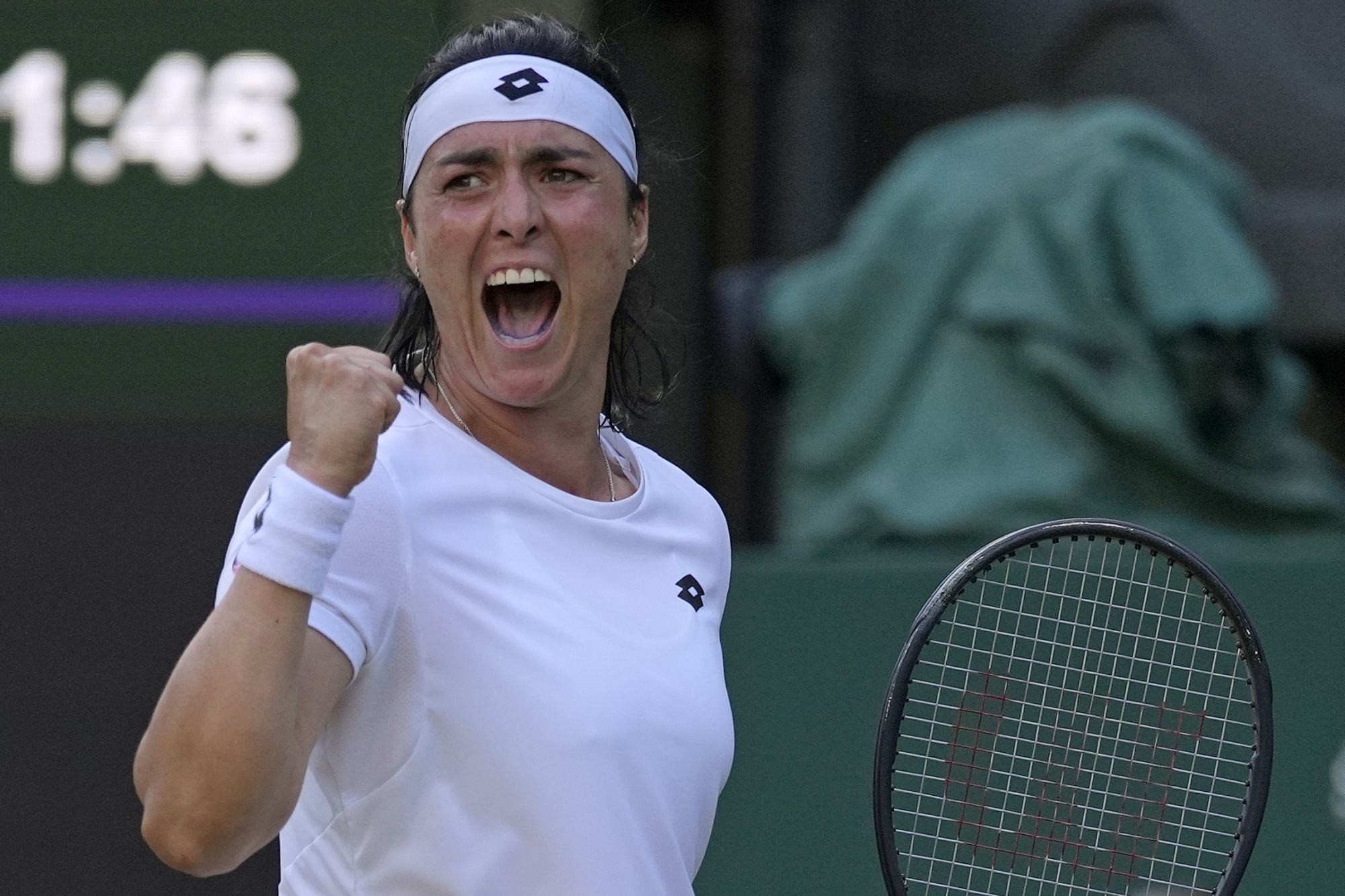An up-close photograph captures Tunisian tennis player Ons Jabeur in a moment of intense celebration. She has her fist raised and is shouting triumphantly, her mouth wide open. Ons is wearing a white short-sleeved shirt, a white wristband, and a white headband, all adorned with a black insignia. She holds a black Wilson tennis racket with a visible "W" on the strings. Her dark black hair and focused expression reflect her exhilaration. In the background, there is a green backboard and a piece of camera equipment covered with a green tarp, which sits on a green stage. To her left, the scoreboard displays the time "11:46" in white font.